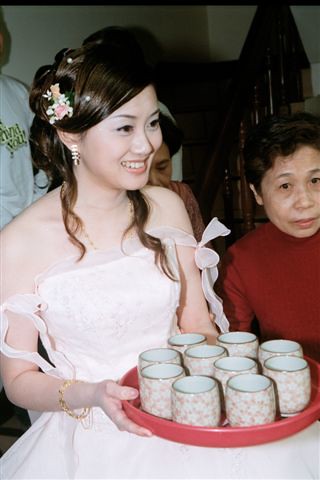In this image, a young Asian woman dressed in a very elegant off-the-shoulder white or pale pink ball gown, possibly her wedding dress, dominates the frame. Her hair is styled in a fancy updo adorned with a peach or pink flower, and she is smiling broadly. She is wearing makeup with pale lipstick and a bracelet on her wrist. The woman holds a round red plastic tray with 13 handle-less cups that resemble mugs. These cups are marbled in various shades of off-white to light brown and have a light green ring around the top edge, with a white interior that could possibly contain some liquid.

To the right side of the woman, an older Asian woman, who could be her mother, is wearing a red turtleneck and looking on with a serious expression. This older woman has short black hair. In the background, there are other people dressed in casual or street clothes, including someone in a white sweatshirt with green lettering. The background appears fairly dark, featuring white walls and some wooden furniture.